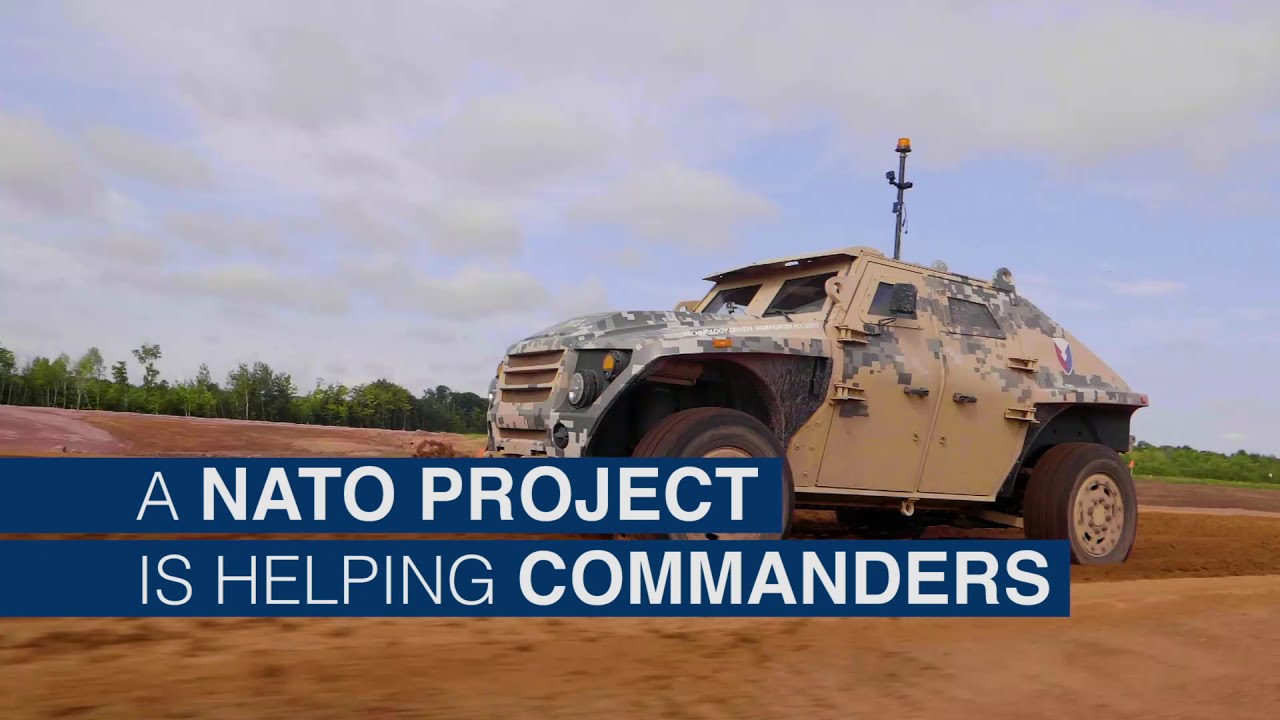The image displays a military SUV, resembling a tan and gray camouflaged Humvee, driving along a reddish-brown dirt road. A tall metal post with an orange light emerges from the roof of the vehicle, which is equipped with large black tires. The setting appears to be an outdoor area with a horizon lined with green trees and bushes. Above, the sky is mostly cloudy with patches of blue. Across the image, a dark blue banner with white text reads, "A NATO project is helping commanders," suggesting this might be a promotional slide or an online photo for a NATO military initiative. The vehicle is slightly off-center to the right, emphasizing the expansive dirt road it travels on.